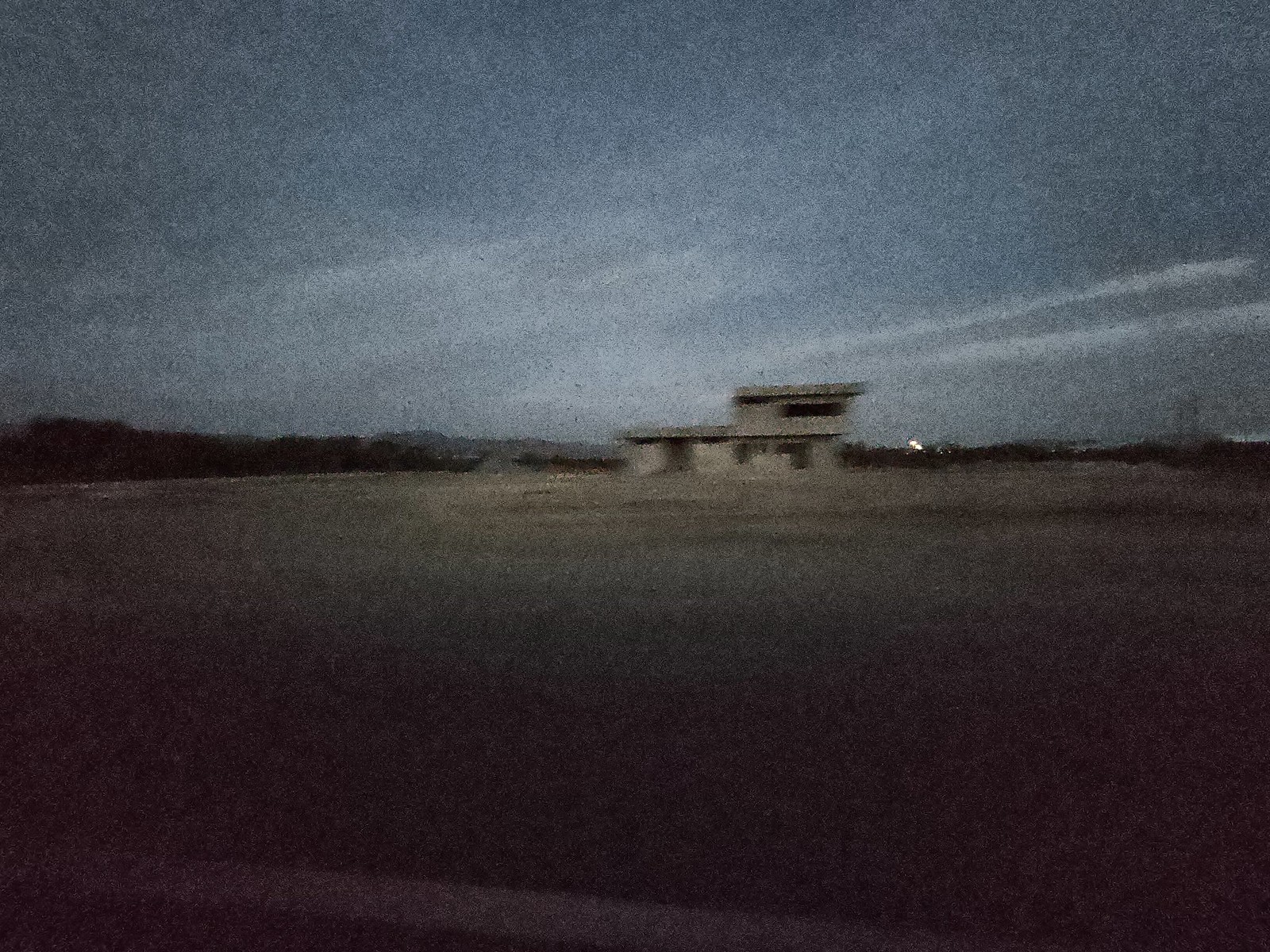This nighttime photograph features a contemporary concrete structure prominently centered in the frame. The building's first level, located on the left side, includes an entrance and two window-like openings. Above, the second floor only partially covers the right side, featuring a long rectangular window and a thickly sloped roof. The greyish taupe structure sits against a background of similarly colored dirt, blending subtly with its surroundings. In the foreground, a roadway is visible, marked by hues of gray and faint white lines. The sky is painted in deep blue tones with notable striations of white, particularly on the right-hand side where two parallel streaks of light cut through the night.